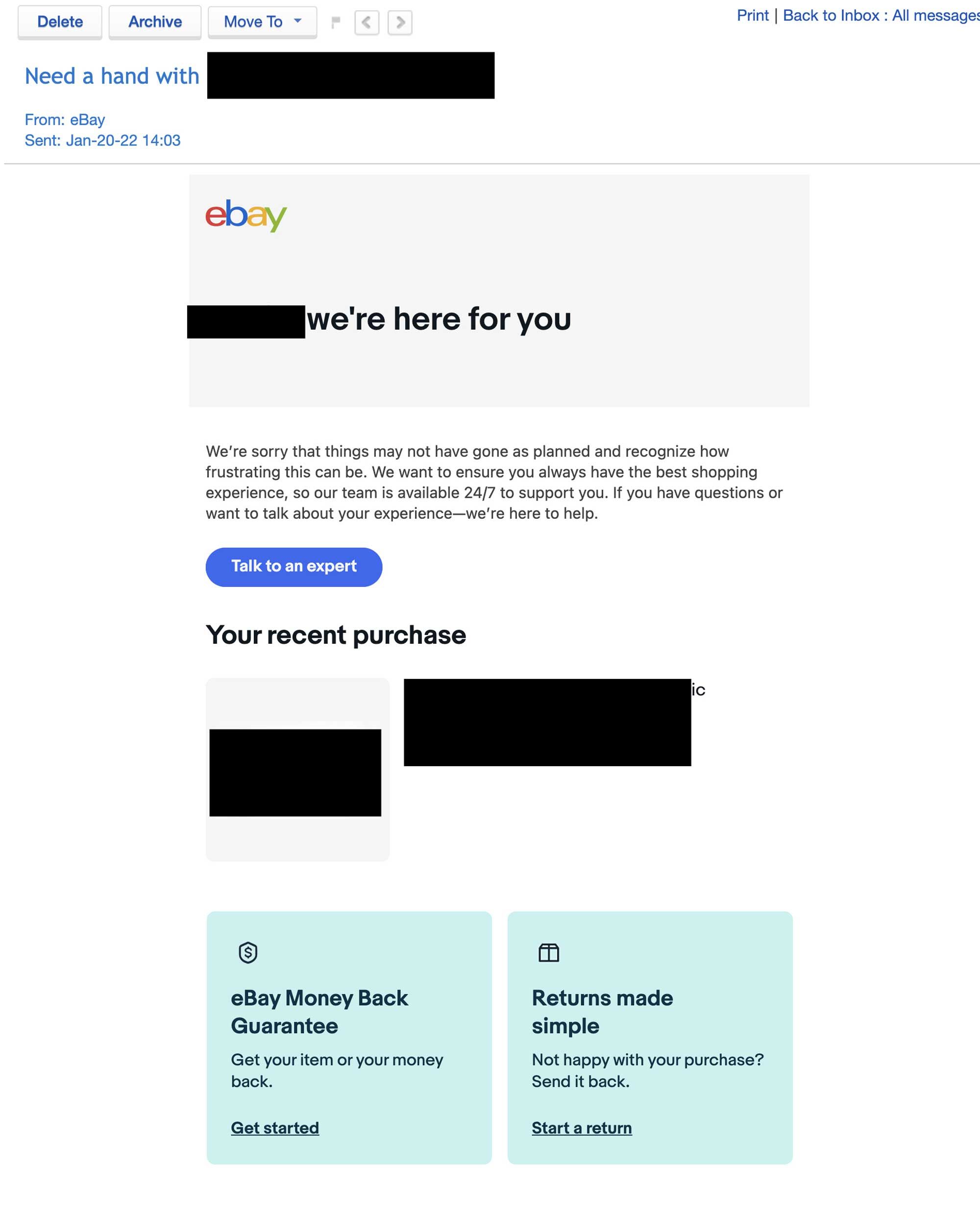The screenshot depicts an email inbox interface, likely from a personal computer. At the top left of the screen, there are three buttons labeled "Delete," "Archive," and "Move to," indicating actions that can be taken on selected emails. Next to these buttons is a small flag icon, along with forward and back navigation buttons.

On the far right corner of the interface, text options read "Print," "Back to inbox," and "All messages," suggesting some navigation and document management features.

The top part of the email itself displays an eBay logo, with a message header that reads: "Blank, we're here for you." The email acknowledges an issue, stating: "We're sorry that things may not have gone as planned and recognize how frustrating this can be. We want to ensure you always have the best shopping experience, so our team is available 24-7 to support you. If you have questions or want to talk about your experience, we're here to help." Beneath this text, there's a "Talk to an expert" button.

The email subject or main content line starts with "Need a hand with," but the rest of the text is obscured by a large black mark. The email notes that it is from eBay, sent on January 20th, 2022, at 14:03.

The lower section of the email contains two blocks of information, though detailed contents are blacked out. The left block features a mint green square with the eBay Money Back Guarantee, accompanied by a shield icon with a dollar sign, and a call-to-action: "Get your item or your money back. Get started." The right block discusses returns, stating: "Returns made simple. Not happy with your purchase? Send it back," alongside a link labeled "Start a return." This section is visually supported by an icon resembling a package.

Overall, this email from eBay aims to provide support and ensure customer satisfaction with clear action-oriented options for addressing issues related to recent purchases.